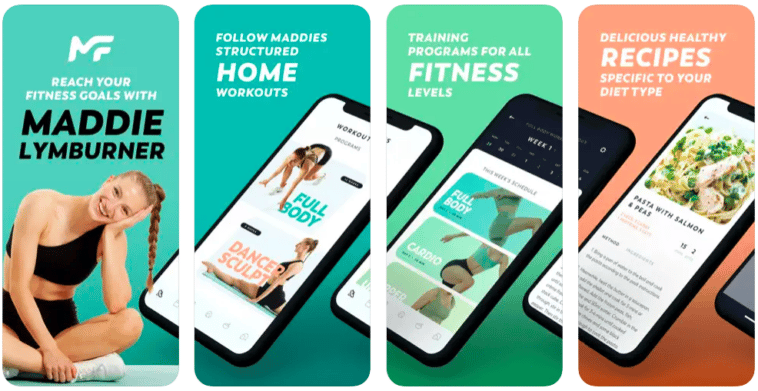The image depicts a series of cascading rectangles, reminiscent of the design style seen on Google or Apple Apps pages. At the forefront, a fit woman sits cross-legged, dressed in a black sports bra and shorts. She tilts her head to the side, resting her right hand against her face. Her hair is a blend of brown and blonde, styled into a braided ponytail, and she wears white shoes.

A prominent logo with the letters "M" and "R" appears against a teal background, alongside the bold, white text "Reach your fitness goals with." Directly beneath, bold black text reads "MADDIE LIMBERNER." A new line presents her name in all caps as "L-Y-M-U-R-N-E-R." Moving within the layout, a mockup of a smartphone partially overlaps this section, transitioning to another area showing her in various exercise poses.

In one section, she is seen bending down with the caption "Full Body" in teal. Another section features her sitting with legs spread, labeled "Dancer Sculpt" in peach. Below this, a darker blue background with white text reads "Follow Maddie's structured," and "Home" in bold white, followed by "Workouts." This section merges into a green rectangle with white text proclaiming "Training programs for all," followed by "Fitness" in bold white and "Levels."

Additional rectangles showcase her in different activities: kicking up with the caption "Full Body" on a teal background, running in a teal sports bra and black shorts labeled "Cardio," and standing partly cut off, wearing a forest green sports bra.

On the right side, a peach background with white text reads "Delicious, healthy," followed by "Recipes" in bold white. It also notes "Specific to your diet type," accompanied by an image of pasta, chicken, and cut-up greens. The bottom part of the image transitions into a darker brown and red mixture.